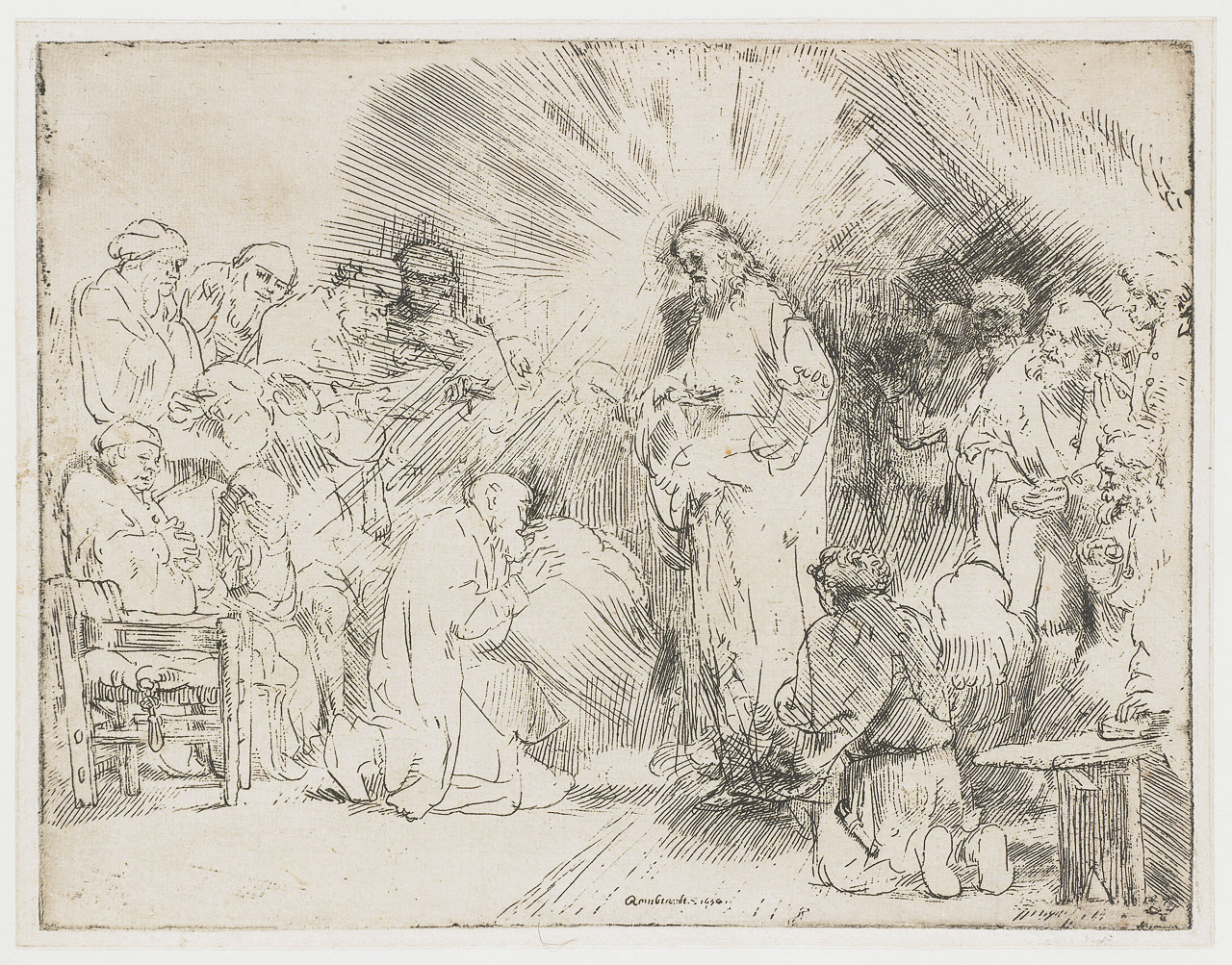This detailed and evocative black-and-white drawing, likely intended for print, features a central figure resembling Jesus, distinguished by a beard, mustache, and radiant lines emanating from his head. The scene unfolds indoors with a dirty white or beige backdrop, contributing to its aged and historical appearance. Jesus stands in the middle, exuding a serene and commanding presence.

Around him, several figures, predominantly older men often with beards and simple clothing, are depicted in various postures of reverence. Two individuals are kneeling directly in front of Jesus, one with hands pressed together in prayer, while others kneel nearby. Several men also stand in observance, some positioned behind Jesus and others opposite him, creating a semicircle around the central figure.

The setting includes sparse furniture, such as a table to the right and what appears to be a bed or couch-type object near Jesus, emphasizing the indoor environment. Despite the detailed sketching, the only visible text lies at the bottom of the image, rendered unreadable due to its diminutive font size. The cumulative effect of the drawing is one of solemn devotion, captured in an intricately sketched, monochromatic style.